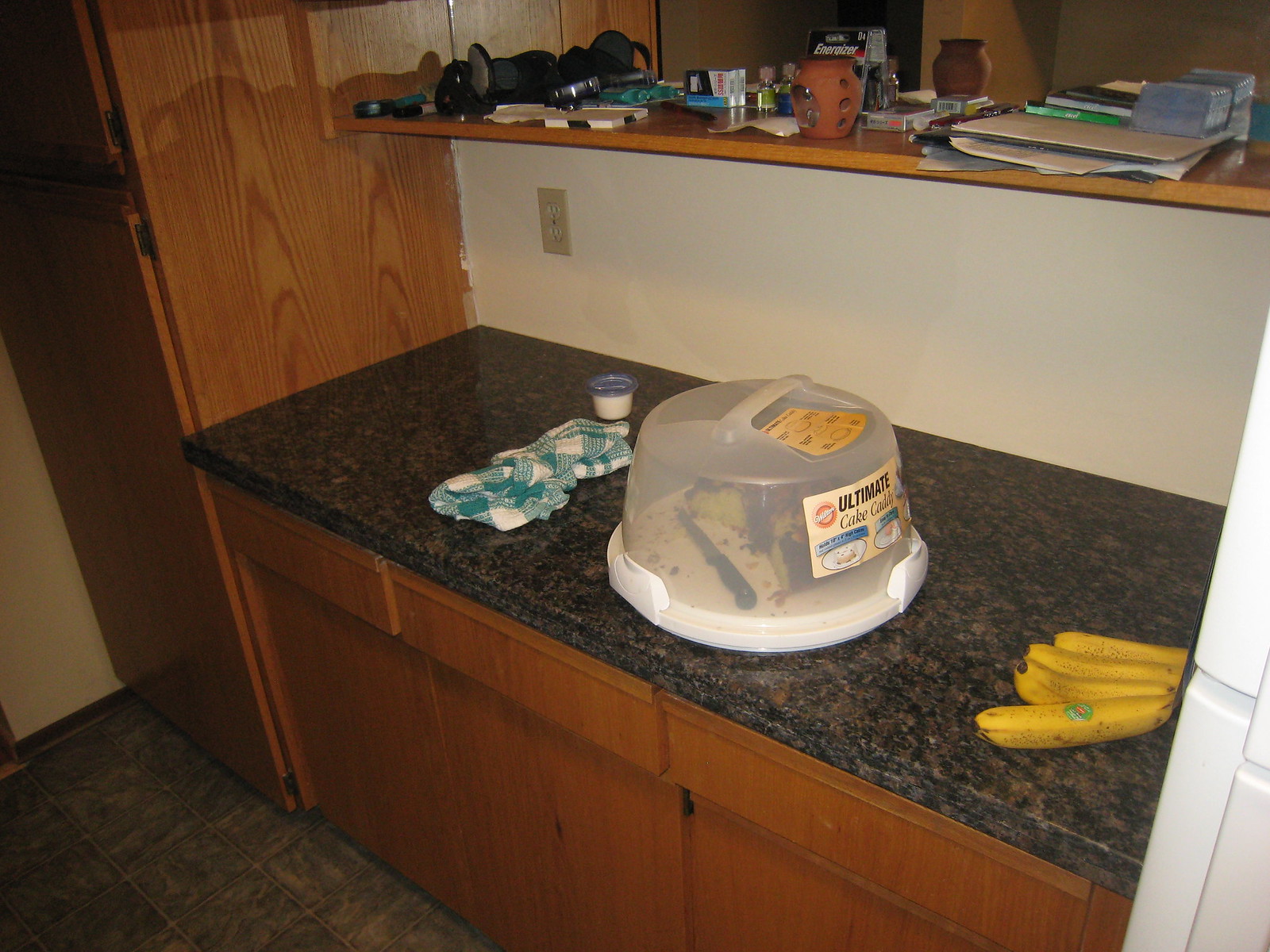**A Detailed Kitchen Counter Description:**

The scene appears to be set inside a home, featuring a countertop that serves as the focal point. The countertop itself is a dark, mottled surface with an interplay of black and brown hues, providing a rich, textured appearance. Surrounding the countertop are light brown wooden cabinets, with the cabinet on the left side extending vertically out of the frame, indicating its considerable height.

Centrally positioned on the countertop is a transparent cake dome, showcasing a cake inside and accompanied by a knife, suggesting a recent or anticipated cutting. To the right of the cake dome, a bunch of four bananas rests casually against the counter. On the left side, there's a green and white rag lying flat, next to a small cup.

In the background, a white wall stands uniformly, interrupted by a double electrical socket situated just below a narrow wooden shelf. This shelf hosts a collection of miscellaneous items: a pack of Energizer batteries, two small orange jars, a blue container, and several books. To the left on the same shelf, a few black objects, likely a pair of headphones and some markers, can be discerned.

Behind these items, the scene recedes into a darker area, possibly another section of the house, creating a contrast with the well-lit kitchen space. Finally, the bottom left corner of the image reveals the flooring beneath the countertop, which consists of grayish tiles, complementing the overall color palette of the kitchen environment.